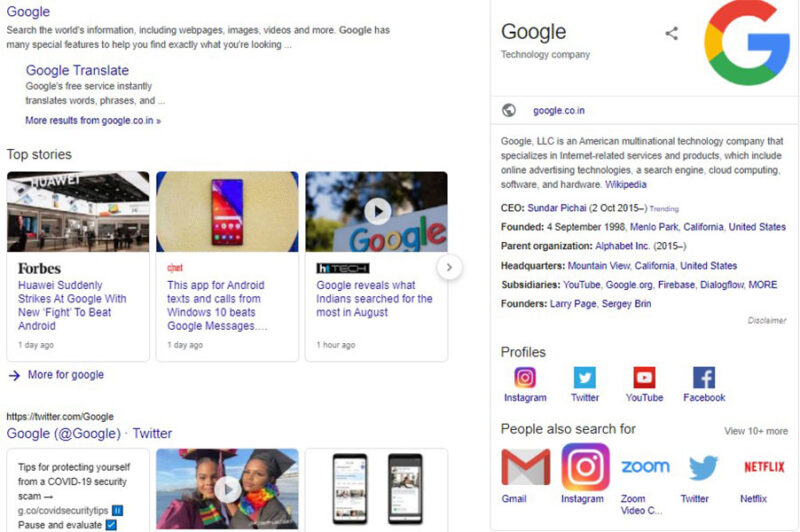The image portrays two versions of a website, demonstrating both desktop and mobile views. On the left side, there is a rectangular layout that likely represents a tablet view. At the top, the page is labeled "Google," followed by a section for "Google Translate" with accompanying text. Below this, a "Top Stories" section displays three photos. The first photo includes a circular icon with a triangle pointing right, indicating a video. The sources for these stories appear to be Forbes, an unreadable text, and a Google-related image, the latter of which directs users to a short video.

To the right, the mobile device view occupies approximately one-third of the overall page. This version is configured in a smaller, more compact format. At the top, the "Google" title appears in a rectangular box, showcasing the iconic red, yellow, green, and blue Google logo. Beneath it, there is a globe icon and a URL, google.co.in. Text below this URL provides a brief overview of what Google is, including details like the company's founding information and CEO.

Further down, there are profile icons for various social media platforms including Twitter, YouTube, Facebook, and Instagram. Below these icons, a section titled "People also search for" lists Gmail, Instagram, Zoom, Twitter, and Netflix, each accompanied by their respective logos. 

This visual effectively compares and contrasts the layout and content presentation of the Google website across different device views.